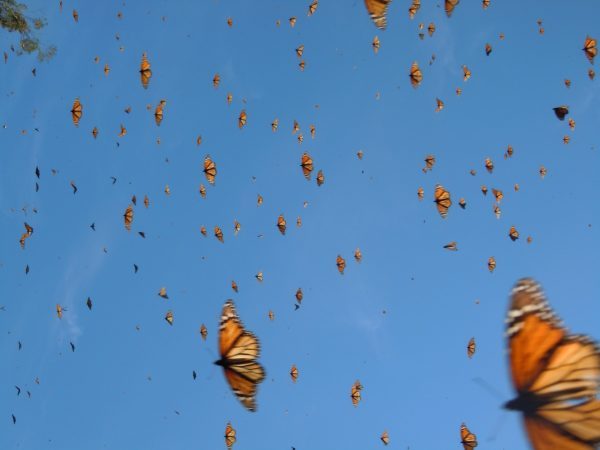The image captures an awe-inspiring sight of hundreds of monarch butterflies in mid-flight, all moving towards the left of the frame. The butterflies vary in size, with the smaller ones scattered evenly across the background and two larger ones prominently positioned in the bottom middle and bottom-right corner, giving a sense of depth and distance. The butterflies are distinguishable by their vibrant orange and light orange wings which feature black veins and borders, along with a sprinkling of white at the tips. This vivid display stands out against a serene blue sky adorned with only a few wispy clouds. In the top left-hand corner, a snippet of a tree branch with green leaves intrudes into the scene, adding a touch of greenery to this skyward view. This photograph, seemingly taken from the ground looking upwards, beautifully captures what appears to be a migration event, showcasing the sheer number and beauty of these monarch butterflies in flight.